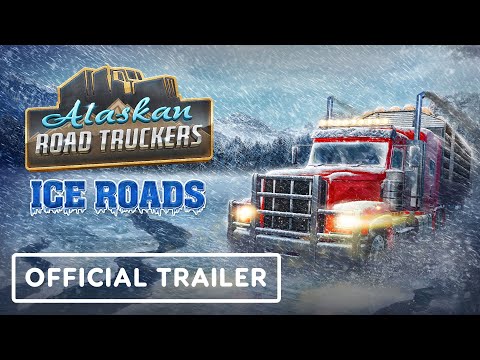The image depicts a vividly illustrated cartoon-like graphic art, featuring a large red semi-truck with a silver frame, trailer attached, and yellow lights, trudging through a heavy snowstorm on an icy, cracked road with water beneath. Beyond the truck, the landscape includes rocky formations and a background of white, gray, and black mountains under a stormy, blue-gray sky. The scene is framed by thick black horizontal bars at the top and bottom of the image, adding contrast. 

In the upper-left corner, the logo "Alaskan Road Truckers" is prominently displayed, with "Alaskan" in light blue and "Road Truckers" in a reflective chrome-like white color, accompanied by an image of a truck's top part. Directly below is the text "Ice Roads" styled in dark blue with icy, frozen embellishments. At the bottom-left corner, a white rectangular box contains the text "Official Trailer" in white font. The overall design suggests an advertisement for a movie or game related to daring truck journeys on perilous Alaskan ice roads.